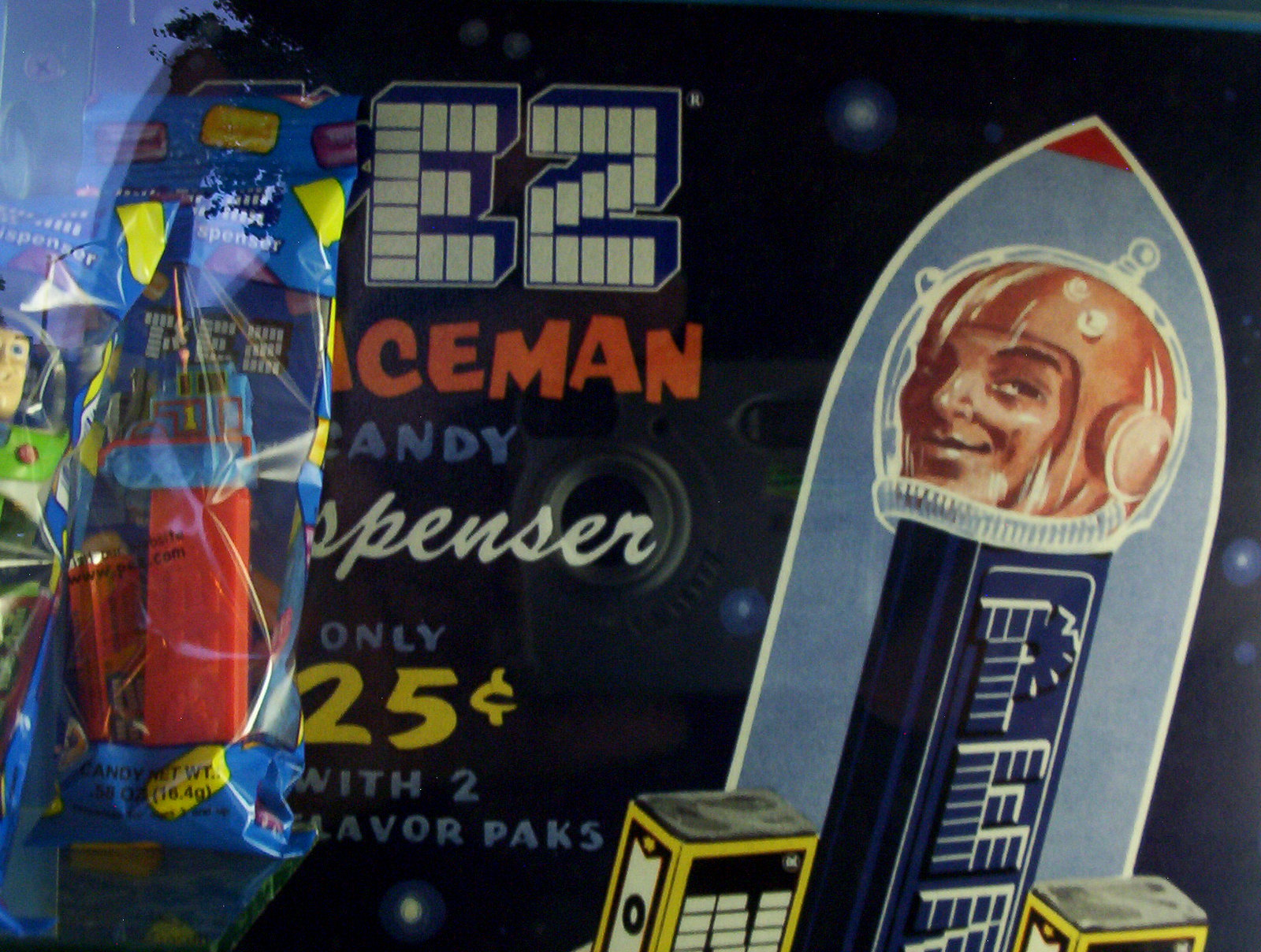The image showcases a vintage Pez candy dispenser advertisement, highlighting a Pez Spaceman dispenser available for only 25 cents, complete with two flavor packs. The advertisement, characterized by a nostalgic design, features a blue-bodied Pez dispenser with a red-helmeted astronaut inside a rocket ship ready for takeoff, set against a starry, space-themed background. The Pez logo stands out in white and blue with "Spaceman" in orange and "dispenser" in cursive white writing. Additionally, the display includes a Buzz Lightyear dispenser and a Thomas the Tank Engine dispenser, both still in their original packaging, visible through what appears to be a glass display.